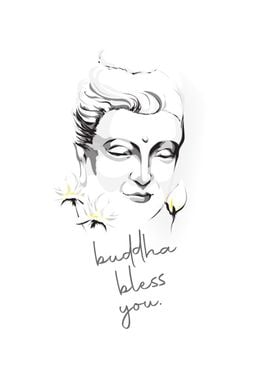This is a small, black and white pencil drawing capturing a minimalist yet evocative essence of a face that appears to be feminine. The illustration focuses on simplicity, using just a few deft strokes to suggest the features and contours. The hair is styled in an updo reminiscent of traditional Buddha depictions, though it can be interpreted as a bun or swept-back style. The eyes are slightly closed, beneath which are a cupid's bow-shaped mouth and a delicate nose. The face is framed by flowers—three roses on either side, tinged with faint hints of color. There is a mark between the eyes, further enhancing its serene yet contemplative aura. Scripted beneath the ethereal visage are the words, “Buddha bless you,” lending a benedictory feel to the piece. Despite its indistinct lines and unshaded areas, the drawing radiates tranquility and grace.